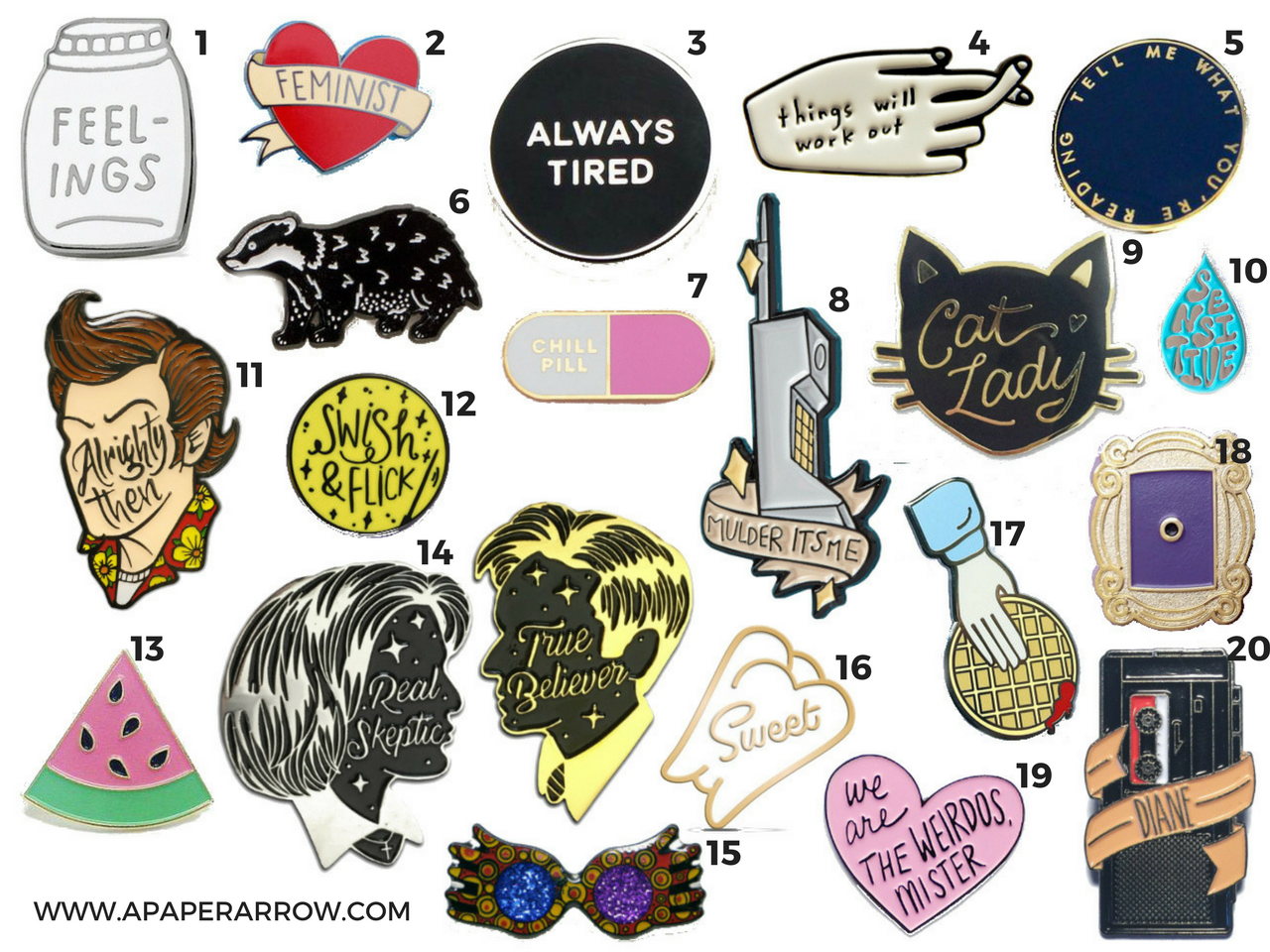This image features an array of 20 eclectic pins or stickers displayed against a white background. Each item is uniquely numbered, and many of them include phrases or images that cater to various interests and subcultures. 

In the bottom left corner, there's a web address, www.paperarrow.com, suggesting these items might be available on this website. Notable items include a gray jar labeled "feelings," a black circle with "always tired" inscribed on it, and a profile of a woman's face with the words "real skeptic." Additionally, there's a profile of a man's face with "true believer" written across it. 

Other intriguing items include a black cassette player marked "Diana," a pink heart with the phrase "we are the weirdos, mister," and a slice of watermelon numbered 13. There's also a vibrant pin resembling a chill pill in pink and white, a cat head with "cat lady," and a pair of wings or hands with purple and blue goggles.

The collection is diverse, with a mix of whimsical illustrations like a tooth labeled "sweet" and expressive phrases capturing feelings and identities. Each item is detailed and thoughtfully designed, showcasing a playful and varied assortment of themes.